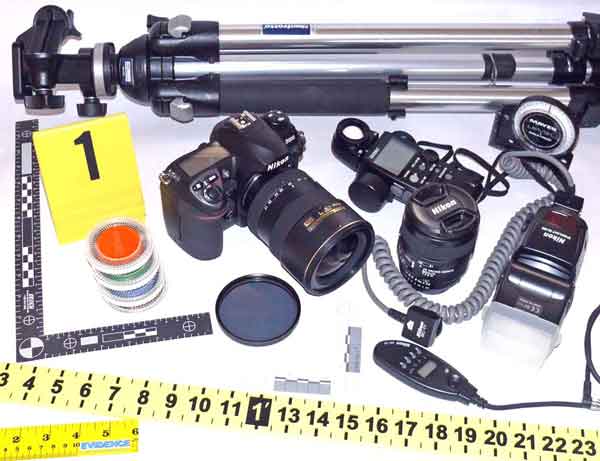The image showcases an array of photography tools laid out methodically. Dominating the top of the image is a tripod, with its silver legs extending from the black top leftwards. Positioned below the tripod is a gray T-square ruler, detailed with measurements and markings. Adjacent to the T-square, a prominent yellow card with a bold, black number one adds a vibrant touch to the collection. Centered in the image is a black Nikon camera, angled with its lens pointing down and to the right. Complementing the camera, a lens cap and an additional lens are situated nearby. Also included in the array are several mysterious black devices with cords and screens, whose functions remain unspecified. Among these, a black flashlight and a yellow tape measure marked with black calibrations can be seen. A peculiar stack of disc-shaped containers sits near the yellow card, enhancing the eclectic mix of equipment. Lastly, a vertical ruler draped across the bottom edge of the image spans from the number three on the left to twenty-three on the right, further emphasizing the organized chaos of the photographic toolkit.